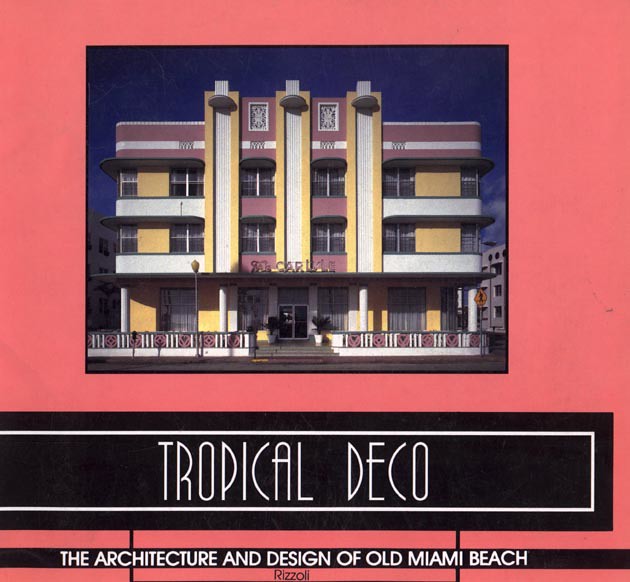The image features a decorative three-story building with a dusty pink, yellow, and white façade, embodying the Tropical Deco style characteristic of Old Miami Beach. The building includes a series of windows on each floor and larger windows at the entrance flanked by potted plants. The front of the building displays gray steps leading up to the entrance, bordered by a uniquely designed railing featuring pink circles. Additionally, there are patios on each floor. Surrounding the building, there are other structures and a road visible in the background. The scene is set against a predominantly pinkish background. Prominently displayed in capital, stylized letters below the building, the caption reads "Tropical Deco" followed by "The architecture and design of Old Miami Beach" on a black horizontal line, with "Rizzoli" written beneath it.